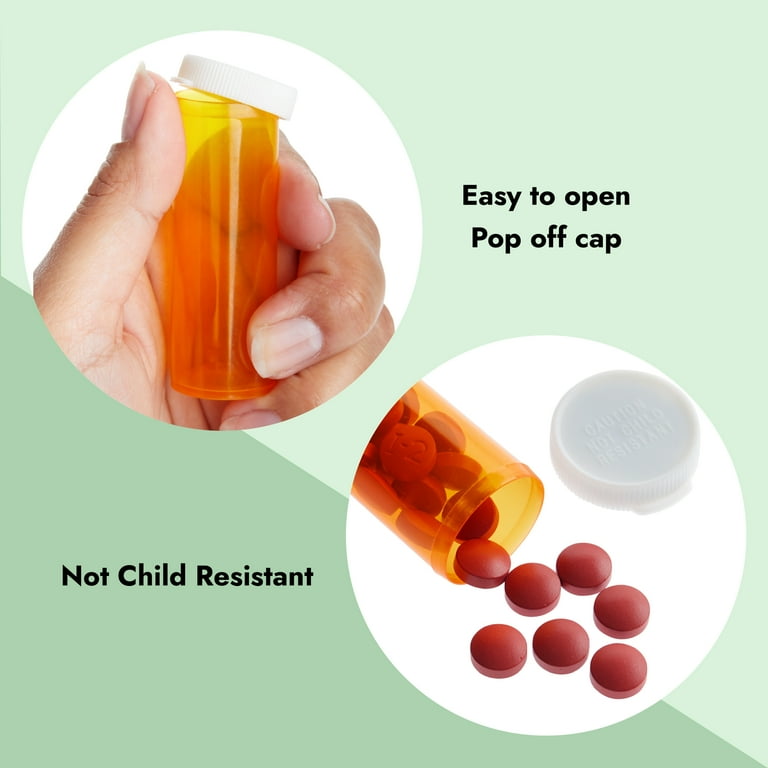The image, likely an advertisement, features a dual-tone green background split diagonally from the top left to the bottom right, with a lighter green segment on the top and a darker green segment on the bottom. In the upper right corner, black text reads "Easy to open, pop off cap," while the lower left corner displays the phrase "Not child resistant" in black text. The ad includes two smaller images with white backgrounds: one shows a well-groomed hand effortlessly removing the cap from an amber-colored prescription bottle using a thumb press, and the other depicts the same bottle with its cap off, spilling red pills onto a white surface. The overall design emphasizes ease of use, particularly for those who may struggle with traditional child-resistant caps.